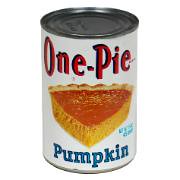This is a detailed photograph of a can of pumpkin pie mix. The can is typical in size, resembling those frequently found in household cupboards. It features a white label adorned with a central image of a delectable pumpkin pie slice, set within a triangle. The upper portion of the label showcases a red graphic that reads "One-Pie" in capitalized, hyphenated text. Beneath this, the word "PUMPKIN" is prominently displayed in blue, uppercase letters. Further down, additional text likely indicating the can's weight or volume can be seen, though it's slightly obscured. The label is designed to be eye-catching and informative, evoking the warm, inviting appeal of a freshly baked pumpkin pie.